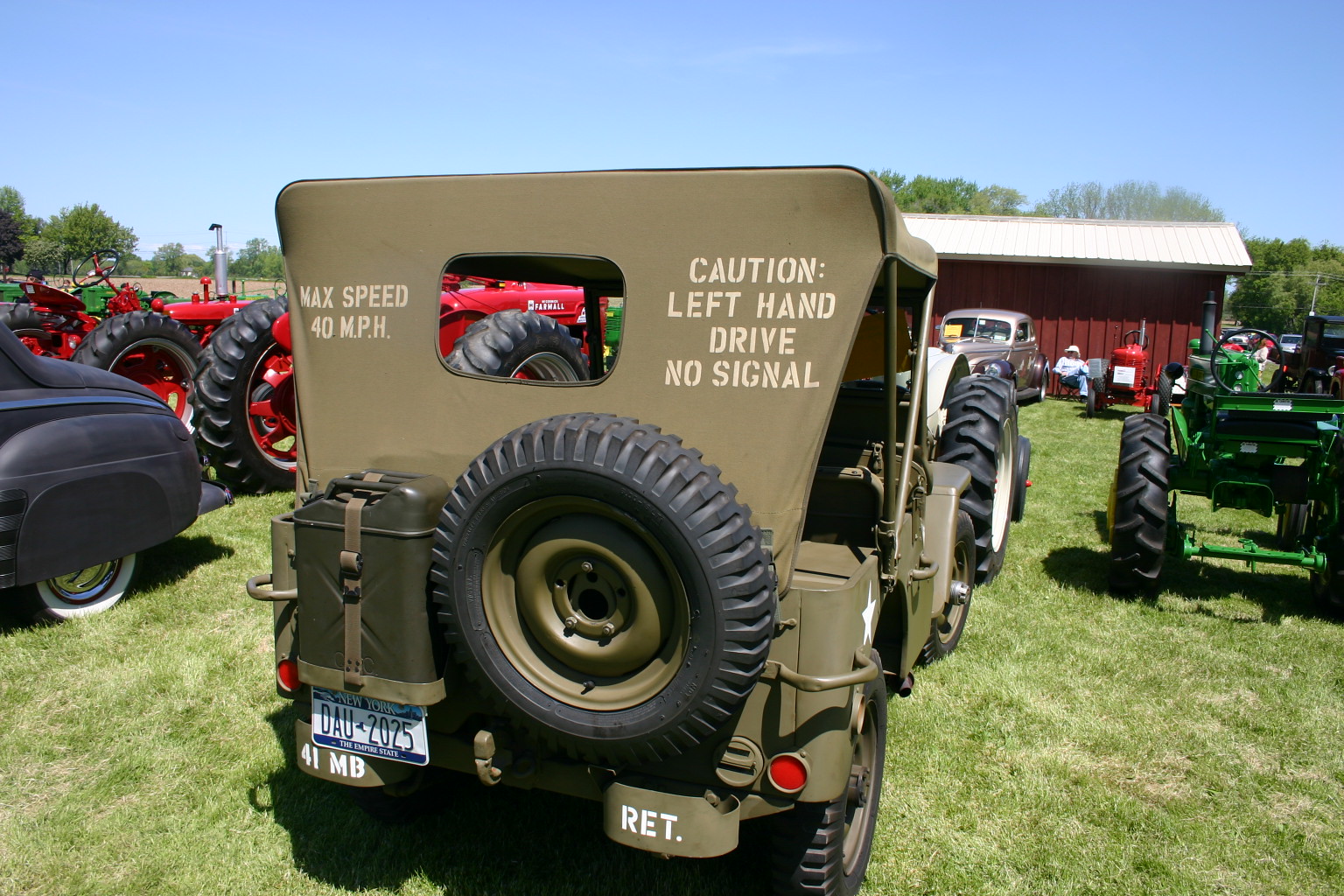In this outdoor photograph taken during a bright, clear day at what appears to be a car and tractor show, a World War II-era Jeep sits prominently at the center. This khaki-colored, open-air Jeep features a large round black tire mounted on the back, beside which a gas tank is securely strapped to the body. The back of the Jeep displays several textual warnings: "Max speed 40 MPH" and "Caution, left-hand drive, no signal." The license plate on the Jeep reads "DAU 2025," and additional markings on the bumper include "41 MB" and "RET."

Set on a lush green grassy field, the scene is populated with various older vehicles and farming equipment. To the left of the Jeep is an old black car, likely from the 1930s or 1950s, recognizable by its white-walled tires. To the right is a small green tractor with black wheels, while further left, a larger red tractor is noticeable. In the distance ahead, there is a red shed with a man sitting on a chair in front of it. The backdrop of the image includes several trees and expansive open fields, all under a blue sky. The overall atmosphere suggests a nostalgic gathering of vintage vehicles and farming apparatus, set amidst a picturesque rural setting.